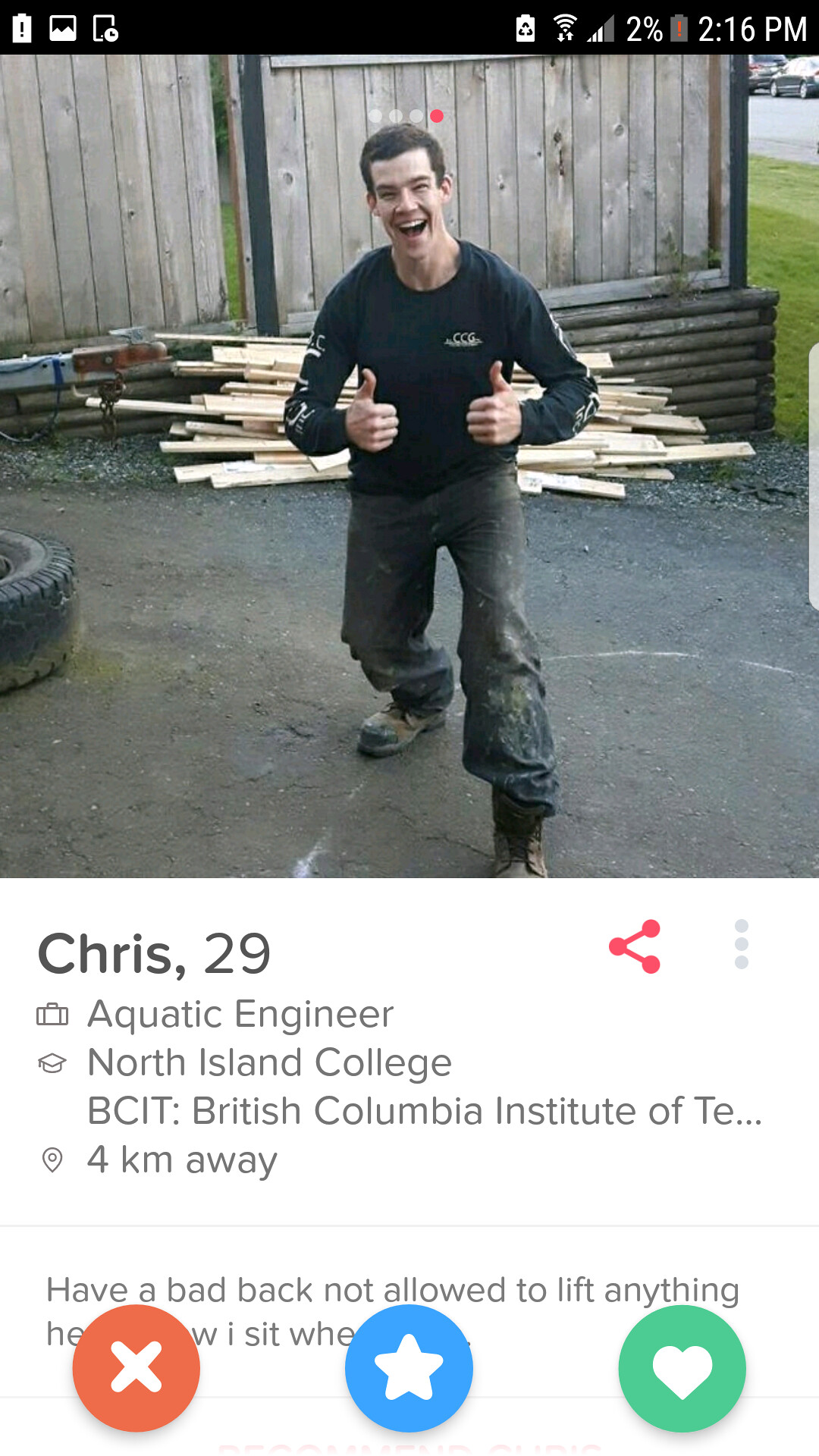The image is a screenshot taken from a cell phone, evident by the black bar at the top showing various icons including cell phone battery life at 2%, a red low battery warning, cellular signal, and the time which is 2:16 p.m. The photo itself features a young man named Chris, 29, an aquatic engineer from North Island College and BCIT, British Columbia Institute of Technology, situated four kilometers away. Chris is standing on a paved surface with pebbles and rocks scattered around, and a large tire is visible to the left side of the image. He is smiling and giving a thumbs up with both hands. He is dressed in a long-sleeved black shirt and dark jeans that are dirt-stained, with one pant leg tucked into his boot and the other over it. Behind him, lumber can be seen, suggesting a construction or work site setting. Additionally, dating profile icons such as an X, star, and heart are present at the bottom of the screen.